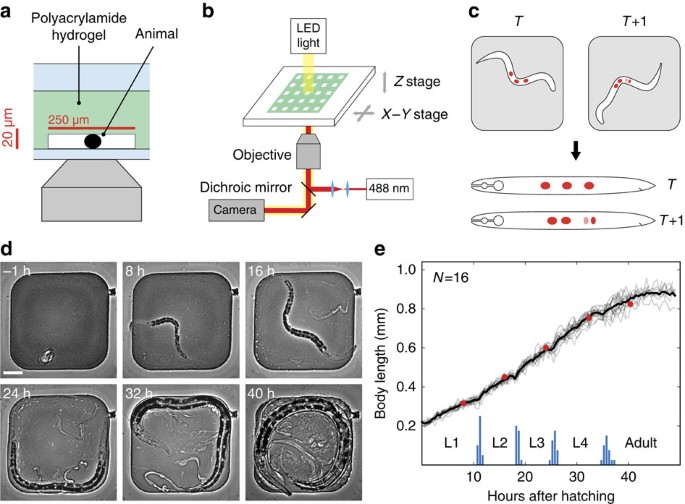This image is a highly technical diagram consisting of multiple labeled sections, arranged in two rows. The top row features sections A, B, and C, while the bottom row includes sections D and E. 

In section A, labeled "Polyacrylamide Hydrogel," a green and blue strip is illustrated, with a line pointing to the green area labeled "Polyacrylamide Hydrogel" and another pointing to a black dot in a white strip labeled "Animal". This section also includes annotations indicating scale dimensions of 250 µm and 20 µm.

Section B depicts a detailed schematic involving an "LED light," a "Z stage" and "X-Y stage," along with components such as an "Objective," "Dichroic Mirror," and "Camera." The notation "488 nm" likely refers to the wavelength of the LED light.

Section C presents two squares containing images resembling worms. The first worm, marked "T," features three red dots, and the second, marked "T+1," features four red dots. Below these squares are two snake-like shapes that correspond to the images above, further labeled as T and T+1.

In section D, located in the bottom left corner, there are six images showing what appear to be developmental stages of worms.

Finally, section E, positioned in the bottom right corner, shows a graph plotting "Body Length" against "Hours after Hatching." The graph tracks developmental stages labeled L1, L2, L3, L4, and Adult, indicating N equals 16.

Overall, this intricate diagram appears to map out experimental data and visualization techniques related to the study of worms, their imaging, and developmental progress over time.